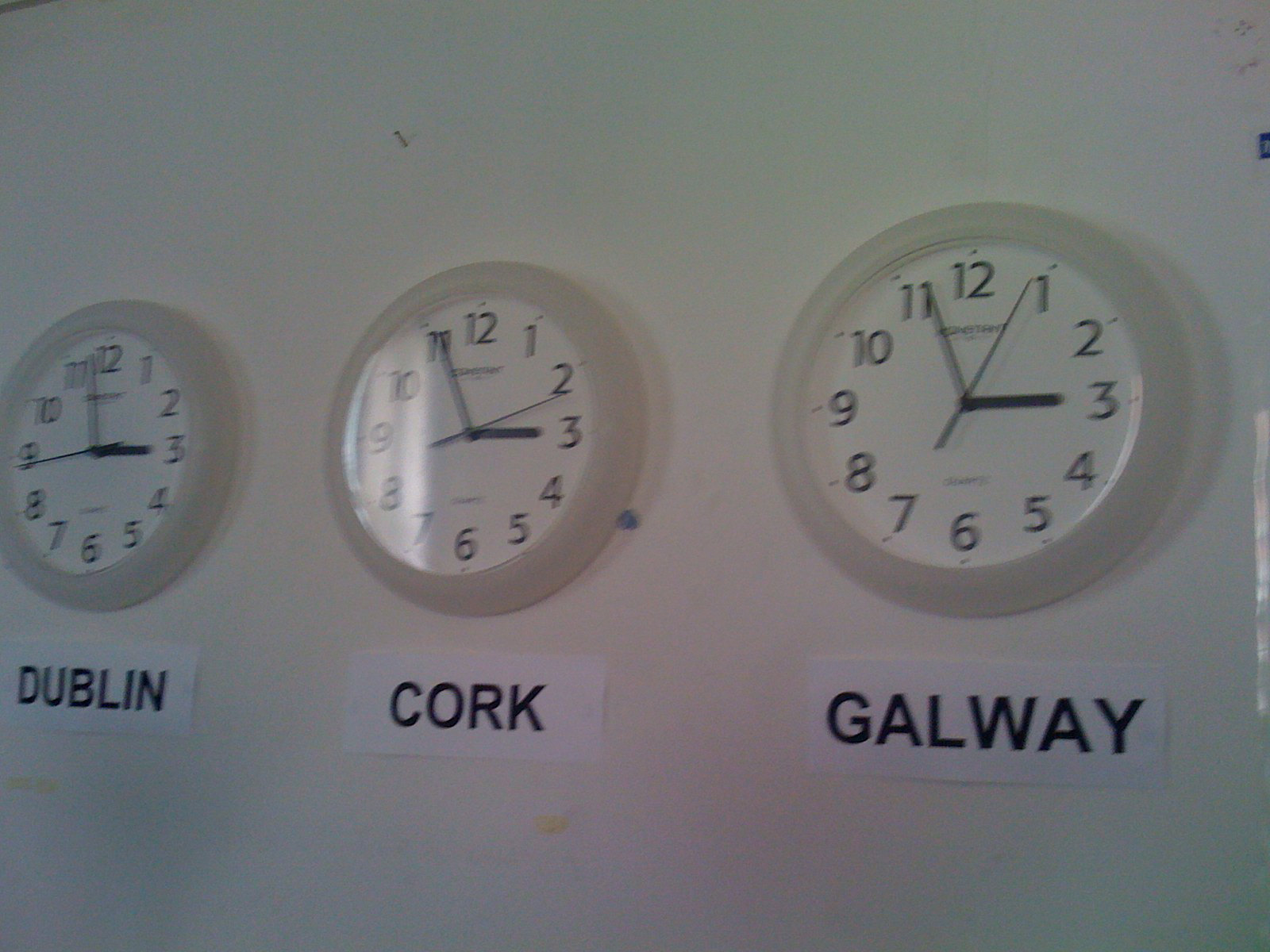In this horizontally oriented and dimly lit amateur photograph, we see three identical wall clocks with white frames prominently displayed against a plain, whitish-gray, and slightly dirty wall. The clocks are aligned horizontally in the center of the image, each labeled beneath with the names of three Irish cities. From left to right, the clocks indicate Dublin, Cork, and Galway. Despite minor variations in the positions of the clock hands—Dublin shows two minutes to three, Cork shows five minutes to three, and Galway shows 2:56 PM—the times are nearly identical, highlighting the lack of significant time difference across Ireland. A small nail can be seen protruding from the wall above the clock labeled Cork.